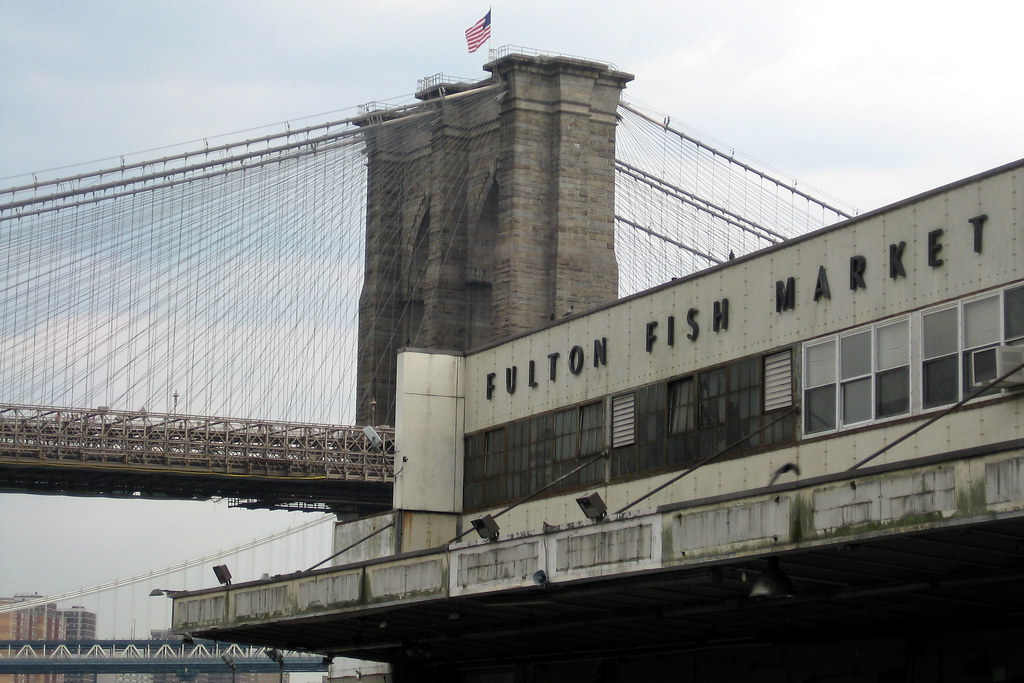This photograph features the dilapidated facade of the Fulton Fish Market, a historic building situated in Lower Manhattan, New York. The light-colored exterior appears washed out and grimy, hinting at years of disuse. The upper floor is adorned with multiple windows, one of which has a room air conditioner sticking out, and a partially visible canopy below them. 

Prominently displayed behind the market is the iconic Brooklyn Bridge, identifiable by its towering structure and the United States flag waving from one of its large pillars. The bridge, built in the late 1800s, adds a majestic historical context to the scene as it spans from Manhattan to the Borough of Brooklyn.

The sky above is pale blue with scattered clouds, giving the photograph a muted, less colorful appearance. In the lower left corner, the faint outlines of distant buildings can be seen, likely part of a housing project either in Lower Manhattan or across the East River in Brooklyn. This setting underscores the urban landscape and the longstanding legacy of the Fulton Fish Market within it.